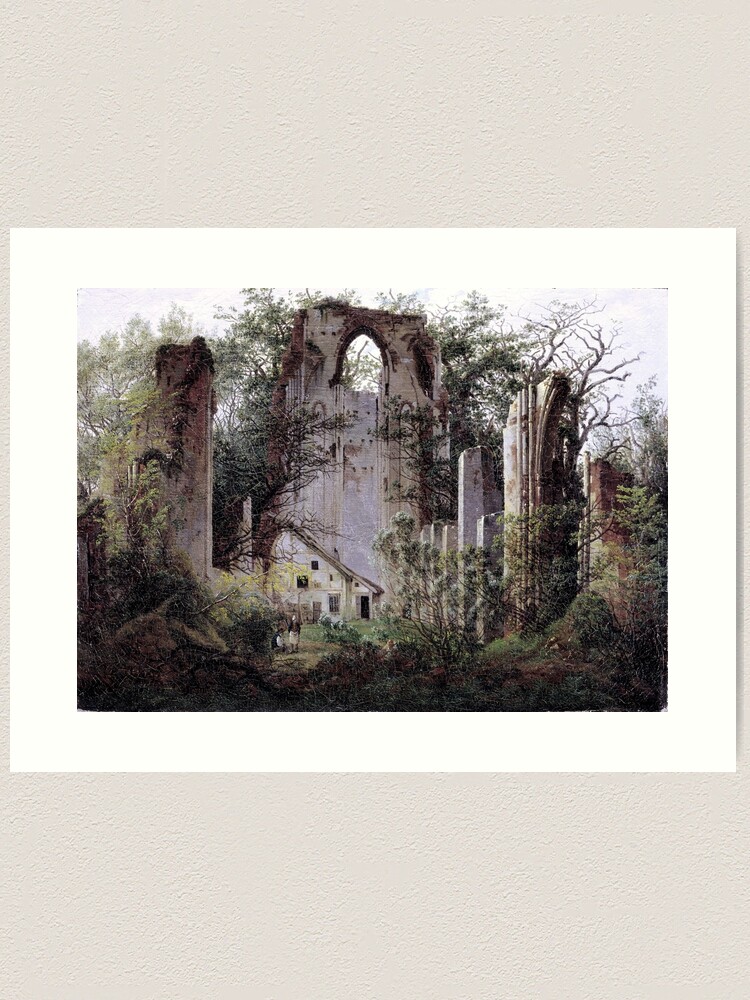The photograph depicts an outdoor scene featuring a large, historic wall that appears to be part of a garden. The wall is gray in color with brown patches, indicating significant degradation and suggesting it is a relic from a long time ago. The structure looks like it could have once been part of a giant cathedral or similar grand building, now overgrown with ivy and shrubbery, lending to its ancient appearance. In the background, through the trees and what seems to be a window in the wall, a small house can be seen, adding to the picturesque quality of the scene. Overhead, the sky is gray and cloudy, enhancing the moody and weathered atmosphere of the photograph.